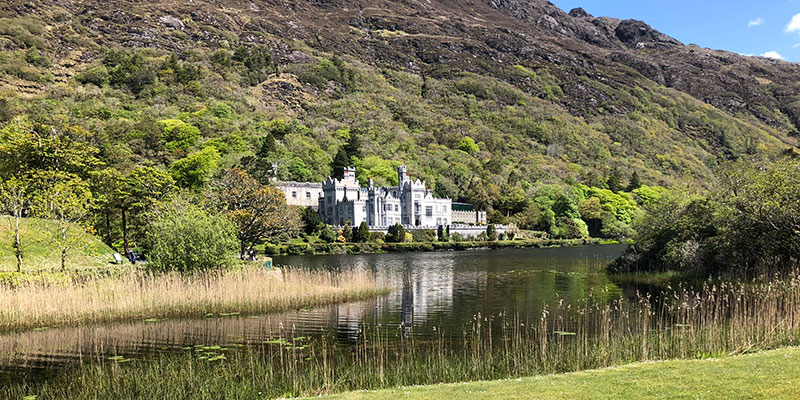The image is a detailed and colorful photograph featuring a castle set against a scenic backdrop. The castle, light gray and presumably made of brick, is nestled at the base of a large mountain. This mountain, covered in lush, bushy greenery at the lower levels, transitions to more sparse and brownish vegetation towards its summit. The sky is visible in the upper right corner, with patches of white clouds against a blue backdrop. 

In the foreground, there's a rippled pond, possibly due to a gentle breeze, with reeds, cattails, and some green lily pads dotting its surface. The water, ranging from dark green to black, reflects the image of the castle, adding a serene quality to the scene. Pale beige reeds and lighter green grasses are present along the pond's edge, consistent with a wetland environment. Overall, the photograph showcases a harmonious blend of greens, grays, blacks, blues, and whites, encapsulating the tranquil beauty of this castle and its natural surroundings.